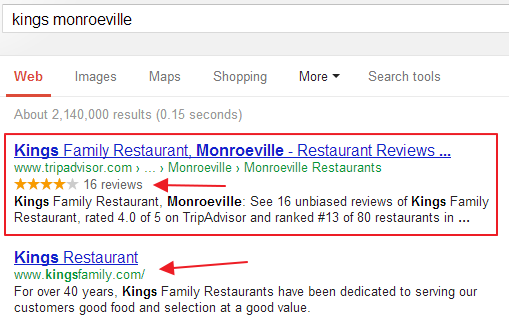In the image, a webpage resembling a search engine is displayed. At the top, there is a white search box containing the text "Kings Monroeville," indicating the search term entered by the user. Below the search box are various navigation tabs labeled "Web," "Images," "Maps," "Shopping," "More," and "Search Tools."

The search results reveal that approximately 2,140,000 entries were found, but only two are visible on the current page. The first search result is for "Kings Family Restaurant, Monroeville," which appears on Tripadvisor. The link, www.tripadvisor.com, leads to reviews specifically for Monroeville Restaurants. According to the brief description, Kings Family Restaurant has received 16 reviews and holds a rating of four stars. It is ranked 13th out of 80 restaurants in the area. This link is highlighted with a red box and features an arrow pointing to the reviews.

The second search result is for "Kings Restaurant" with the website www.kingsfamily.com. The description under this link states that for over 40 years, Kings Family Restaurants have committed to providing good food and variety at a reasonable price. An arrow points to the kingsfamily.com link, drawing attention to it.